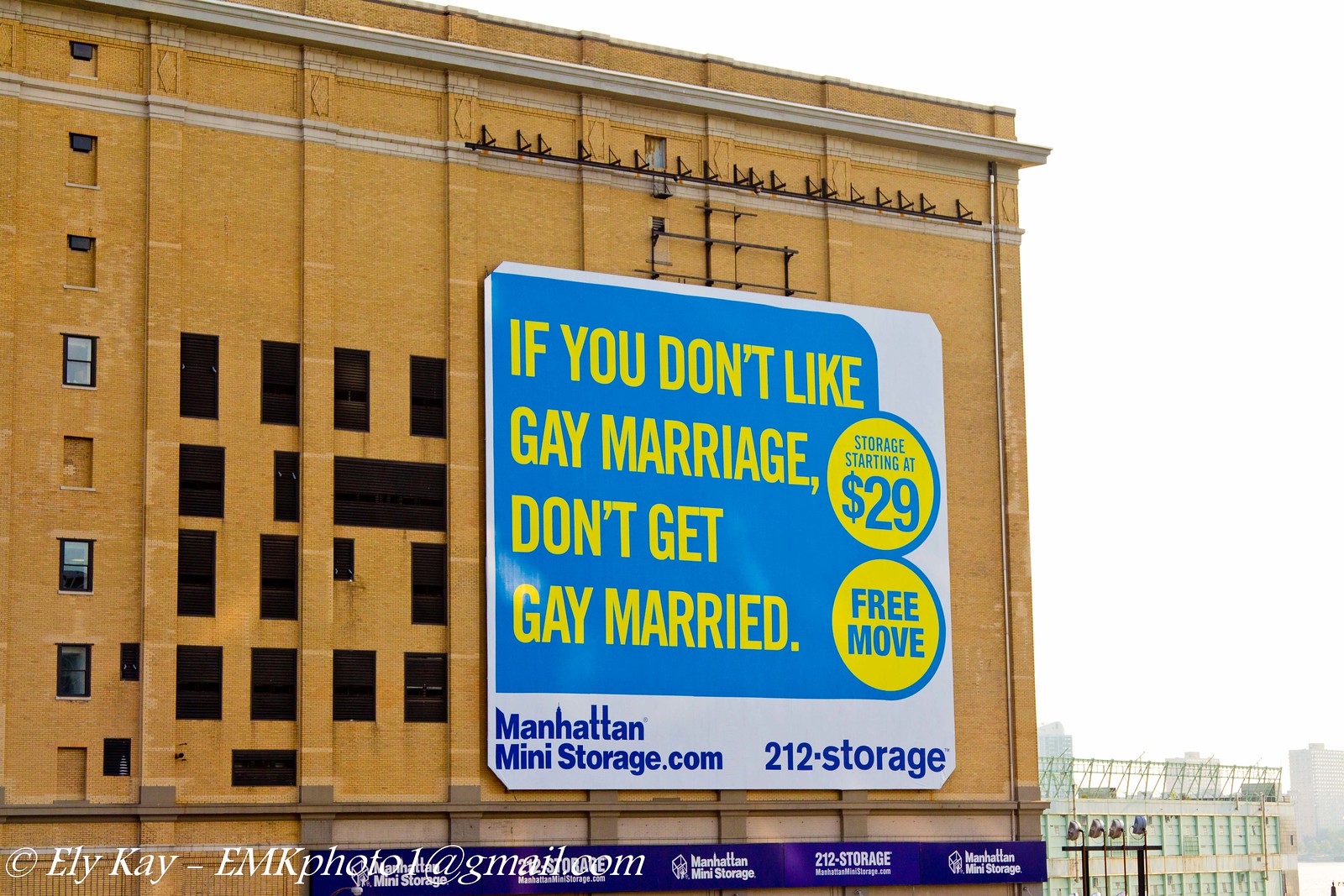The image captures an angled view of the facade of a towering yellow brick building, which appears to be abandoned. The building features numerous small, black-coated windows in the center, while a vertical line of smaller windows on the left side are partly boarded up. Dominating the right side of the building is a large, conspicuous billboard with a white background. The billboard features a substantial blue square overlay, with the bold yellow text proclaiming, "If you don't like gay marriage, don't get gay married." Adjacent to this message, two yellow circles display additional information in blue font. The top circle announces "Storage starting at $29," and the bottom circle states "Free move." At the bottom left of the billboard, the website "manhattanministorage.com" is displayed, while the bottom right includes the phone number "212-Storage." Spanning from the center to the right at the very bottom of the image is a banner repeating the Manhattan Mini Storage logo and contact number. The photo credits are marked at the bottom left with a watermark labeling "copyright Eli K" and an email address "elikemkphoto@gmail.com". The photograph appears to be taken during the day, emphasizing the bright colors and the intricate details of both the building and the advertisement.